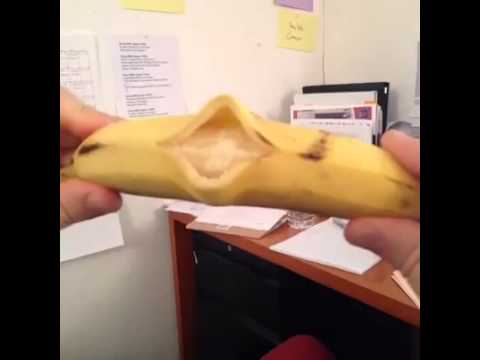The image depicts a work or home office environment with a focus on a banana being held horizontally by two hands. The banana, yellow with some brown spots, has its peel split open in the middle, giving the appearance of a mouth. The left hand holds the left part of the banana, while the right hand holds the right part, pushing the peel upward and downward. Behind the banana, there is a brown wooden desk with white papers scattered on it. The background shows walls with various pieces of paper, clipboards, a black binder, and sticky notes in yellow and purple. The wall is a cream color, adding to the office ambiance. Additionally, the image is framed by two black columns, and a red chair is partially visible.